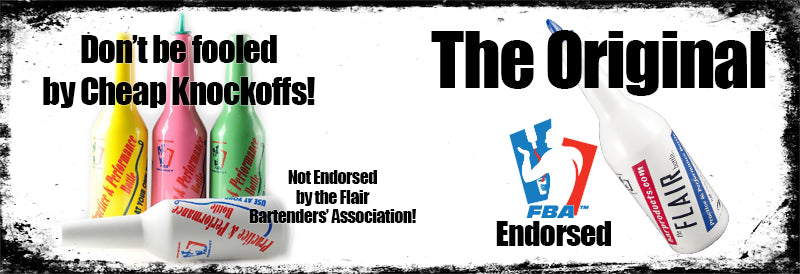The image is a detailed advertisement for the original Flare bottle, shaped longer than it is tall, accented with a black, grungy border. The focal point on the left side showcases four bottles, three standing upright in yellow, pink, and mint green, while a fourth white bottle lies horizontally at their base. Above these bottles, the text warns, "Don't be fooled by cheap knockoffs." Each bottle bears the label "practice and performance bottle," though the text is somewhat difficult to discern.

Moving to the right side, prominently, the text declares "the original" next to a white Flare bottle, which features red, blue, and black text on it. Despite a website address on the bottle being blurred and unreadable, another significant detail on the right is the FBA endorsement, demonstrated by a clip art image similar to the Baseball Association logo, featuring a bartender in white relief against blue and red backgrounds, pouring liquid into a small cup.

In the central section of the ad, there is an apparent contradiction: the text reads, "Not endorsed by the Flare Bartenders Association," juxtaposed against the FBA endorsement symbol on the right side. This conflicting information, coupled with the vivid imagery and varied text placements, might hint at either a clever or confusing marketing strategy, but it reinforces the authenticity of the "original" Flare bottle amidst possible knock-offs.